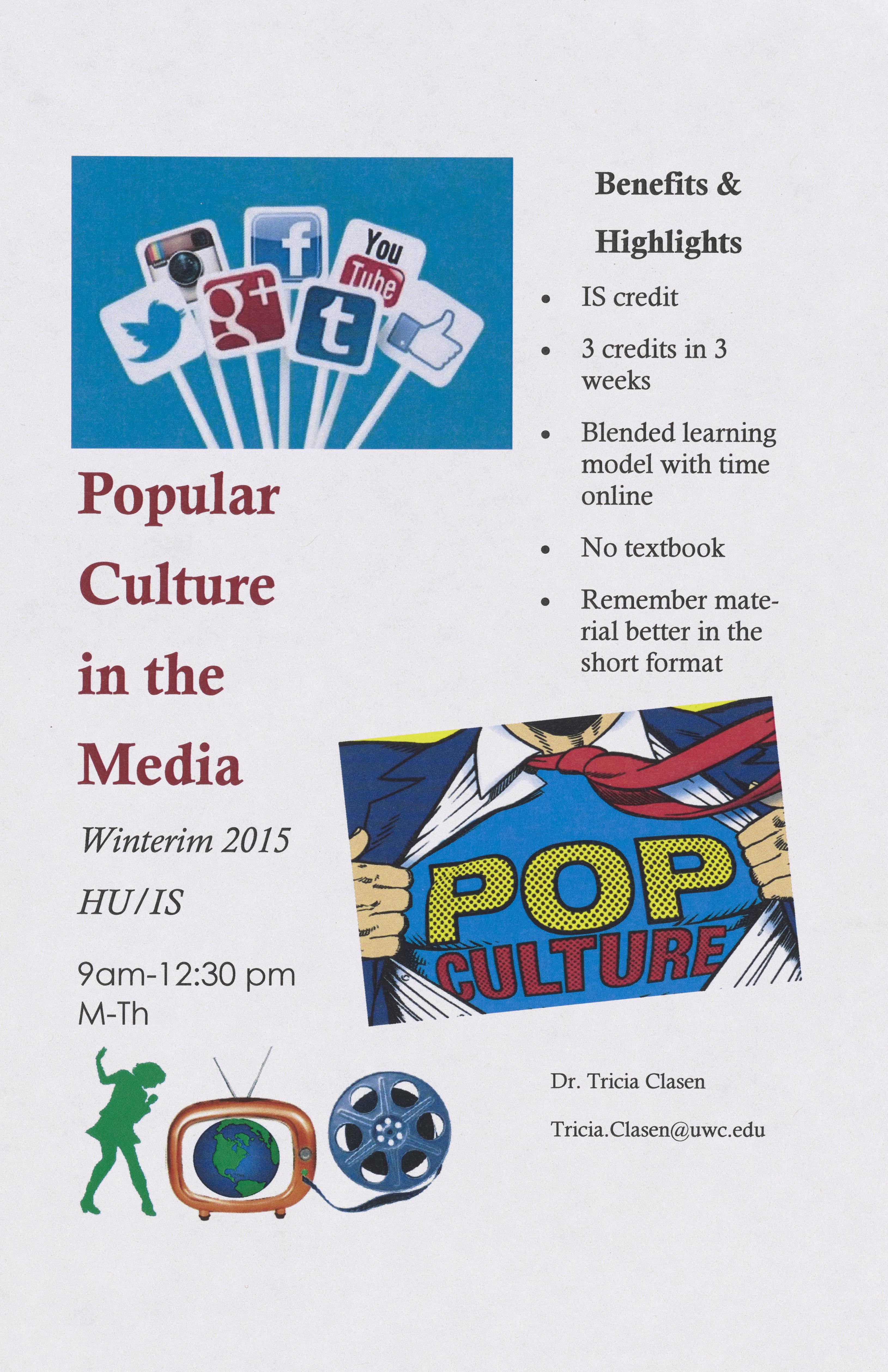This poster advertises a college course titled "Popular Culture in the Media," taught by Dr. Tricia Klassen, and scheduled for Winterim 2015. The course runs from 9:00 AM to 12:30 PM, Monday through Thursday, offering IS credit and allowing students to earn three credits in three weeks. Emphasizing its benefits, it features a blended learning model with online components, no required textbook, and a format designed to help students retain information better through its short, intensive structure. At the center of the poster is an image of Superman ripping open his suit to reveal the words "Pop Culture" on his chest. Social media icons like Facebook, Instagram, Twitter, Google, and YouTube appear prominently at the top, reinforcing the course's focus on media. Additional highlights and benefits are bullet-pointed on the left side, while to the right, there's Dr. Klassen's email (tricia.klassen@uwc.edu) for further contact. The poster also includes vibrant icons of a green dancing girl, a retro television with a globe, and a film reel, adding visual appeal.